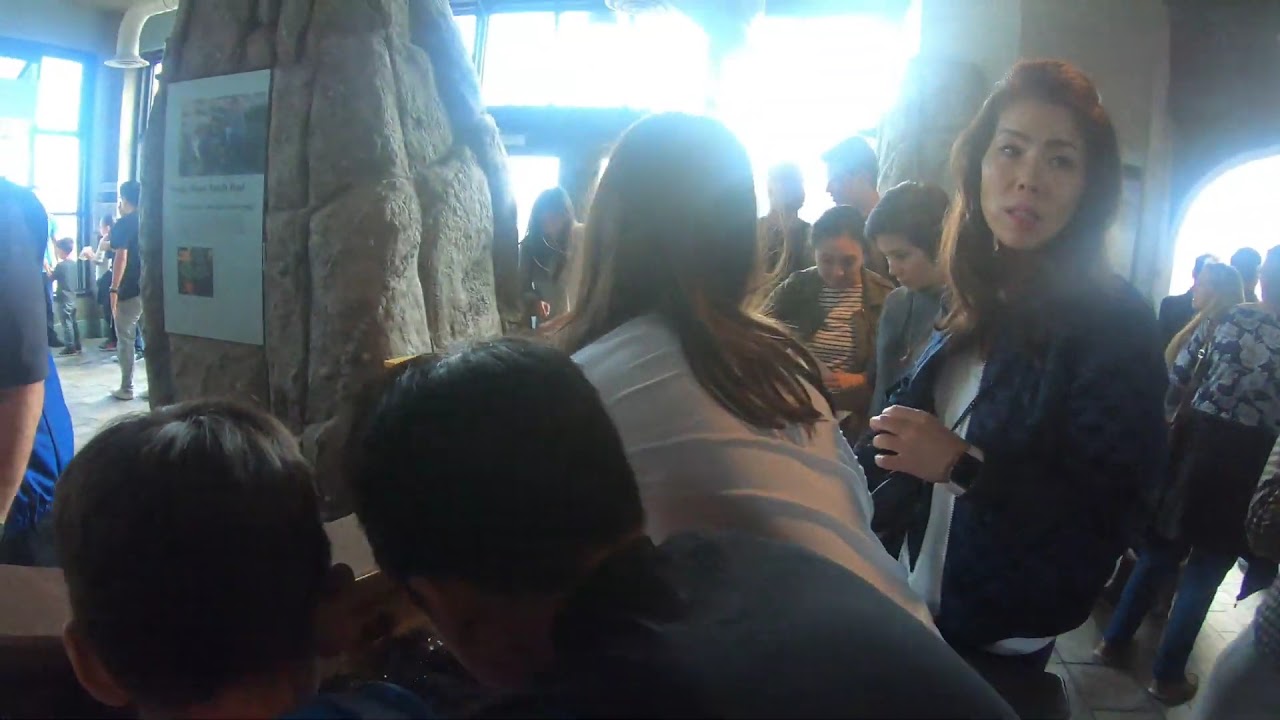The photo captures a bustling scene within a well-lit indoor space, possibly a museum, filled with a large crowd of people congregating around an artificial stone monument adorned with a plaque. The stone is positioned on the left side of the image, with the plaque facing left. The room is bathed in sunlight filtering through windows at the top center, casting a bright glow and slightly obscuring the faces in the crowd. Among the predominantly dark-haired individuals, a woman stands out on the right side, looking back at the camera; she appears to be Asian, clad in a dark blue jacket, and holding a camera. The crowd includes many people leaning in towards the stone, closely examining it or the items in front of it, creating a dense and engaged atmosphere. The scene is bustling, with people spanning from the bottom left to the upper right of the image, highlighting the area’s popularity and sparking a sense of curiosity about the stone's significance.